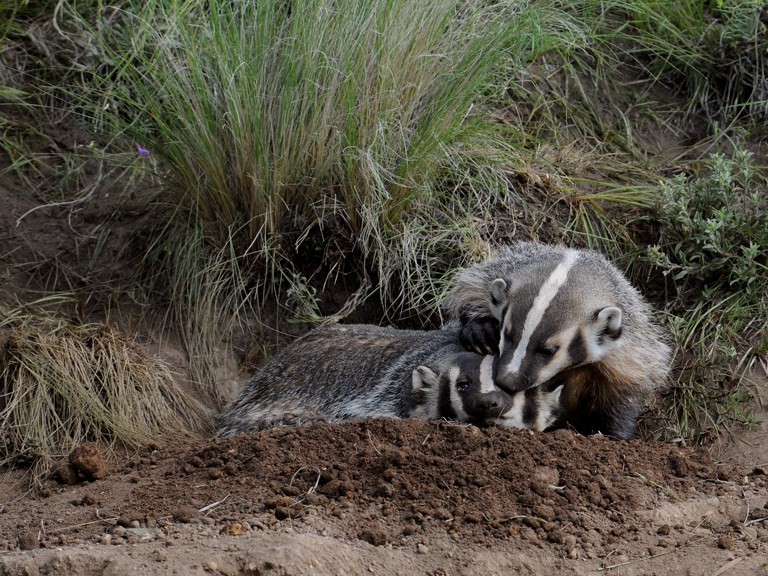This color photograph captures a serene nature scene featuring two adult badgers nestled in a muddy, soil-rich burrow. The badgers, with their dark grayish-brown fur accented by distinctive long white stripes that extend over their heads and down their backs to their snouts, are positioned prominently in the center of the image. One badger lies flat on its stomach while the other endearingly lays on top, gently nuzzling and perhaps even "kissing" its companion. Their cute black eyes and small ears add to their charm as they snuggle together, evoking a sense of companionship and contentment. The foreground is dominated by the earthy, muddy environment they've burrowed into, while the background features a mix of green grass and patches of burnt, straw-colored grass, hinting at the wild habitat these creatures call home. There are no other animals or text, keeping the focus solely on the affectionate pair of badgers and their tranquil surroundings.